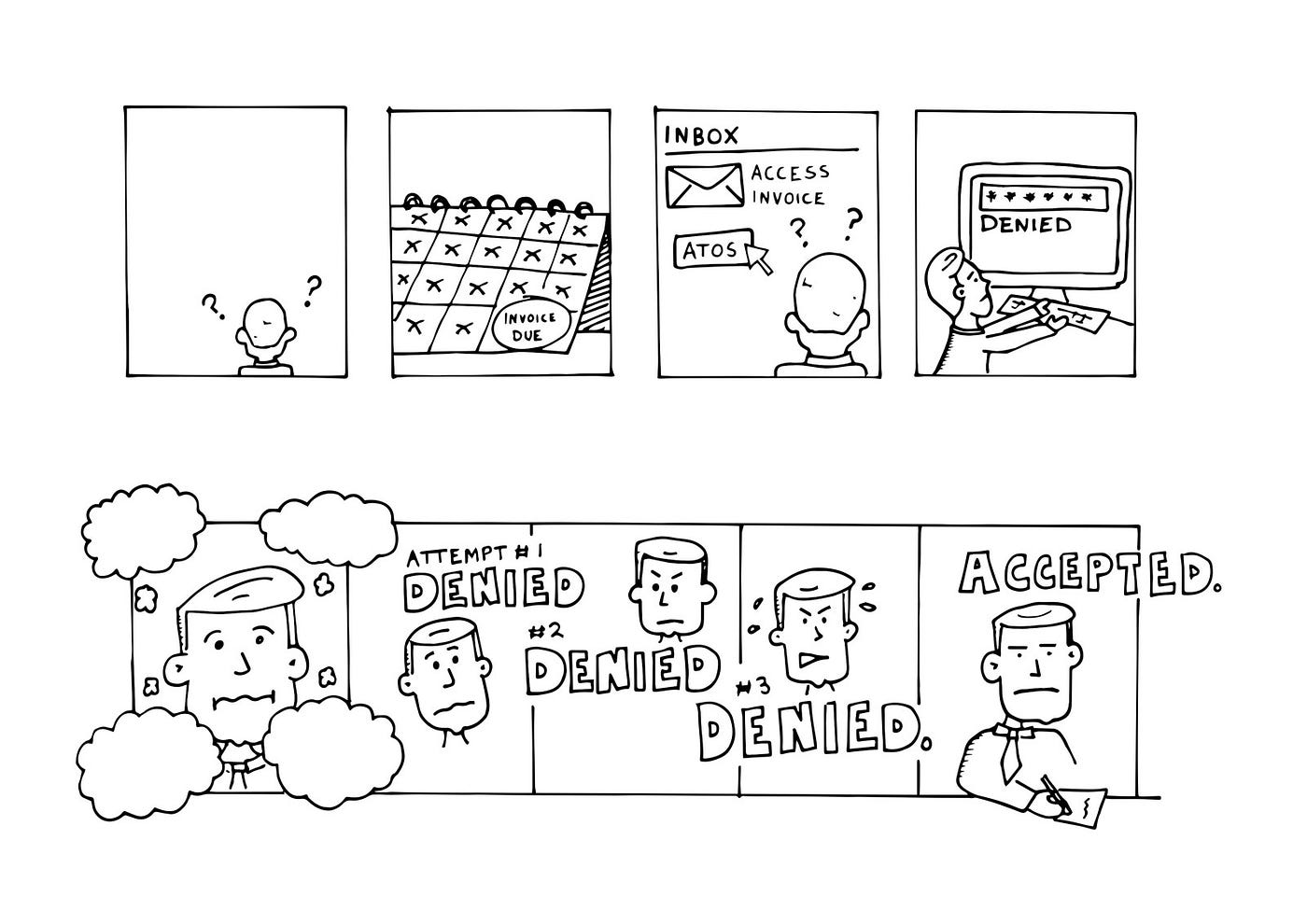This black and white hand-drawn comic strip consists of nine panels. The first panel shows the back of a man's head with question marks surrounding it, indicating confusion. In the second panel, a desk calendar displays all days marked off with Xs except the last one, which is circled and labeled "Invoice Due." The third panel depicts a computer screen with the text "Inbox Access Invoice," an envelope icon, and a box labeled "ATOS" with a cursor pointing to it, again with question marks above the man's head. In the fourth panel, the same man is shown in profile typing on a computer, with the screen displaying a large "Denied" message.

The fifth panel captures the man facing the viewer, appearing frustrated, surrounded by four empty thought bubbles, suggestive of his mental turmoil. The next three panels show a progressively angrier depiction of the man, with text indicating "Attempt 1 Denied," "Attempt 2 Denied," and "Attempt 3 Denied." Finally, in the last panel, the man, now wearing a tie, is seen writing on a piece of paper with the word "Accepted" prominently at the top.